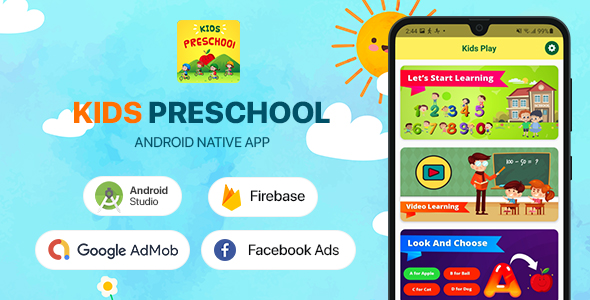This promotional poster is designed to showcase the "Kids Preschool Android Native App". The vibrant, colorful background, featuring a cheerful sky with playful clouds and a smiling sun, caters to children and their parents. On the right side of the poster, a graphic of a mobile phone displays the app’s interface. The app interface highlights activities such as "Let's Start Learning," which features numbers and kids in front of a school, "Video Learning," depicting a teacher in a classroom scene, and "Look and Choose," which uses visual aids like the letter 'A' and an apple for learning.

On the left side of the poster, the app's logo is prominently displayed at the top--a yellow and green square with the words "Kids Preschool" and graphics of children riding bikes across hills with an apple-shaped sun. Underneath the logo, there are icons representing access through Android Studio, Firebase, Google AdMob, and Facebook Ads, indicating the app's integration with these platforms.

Overall, the design aims to attract young learners and their guardians by emphasizing educational content through an engaging and colorful interface.